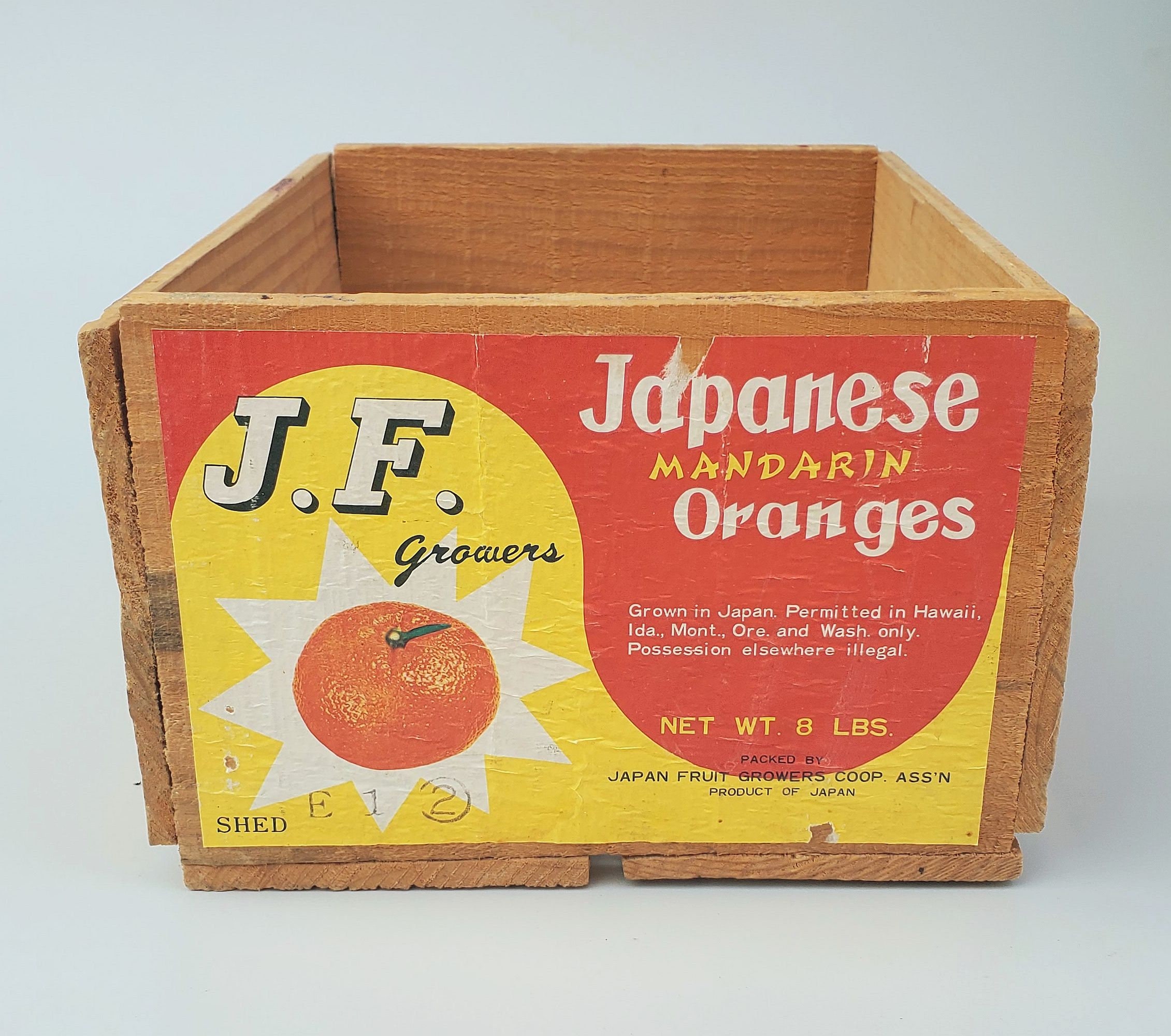This image displays an old wooden crate, likely crafted from reclaimed or pallet wood, exhibiting a brownish-orange hue and appearing to be on the verge of coming apart at the seams. The front of the crate prominently features a large, eye-catching label that is divided into red and yellow sections. Within the red section, the text reads "Japanese Mandarin Oranges" in an oriental-style font. Below, in the yellow section, it states "J.F. Growers," accompanied by the phrase "grown in Japan." Central to the label is a striking image of a mandarin orange encircled by a white star. Further details on the label specify that the oranges are permitted only in the states of Hawaii, Idaho, Montana, Oregon, and Washington, noting that possession elsewhere is illegal. The net weight of the crate is listed as eight pounds, and the produce is packed by the Japan Fruit Growers Co-op Association, marking it as a product of Japan. The sides of the crate, assembled with nails, seem to be pulling away slightly from the main structure. Additional wood pieces at the bottom provide extra height and stability to the old crate.